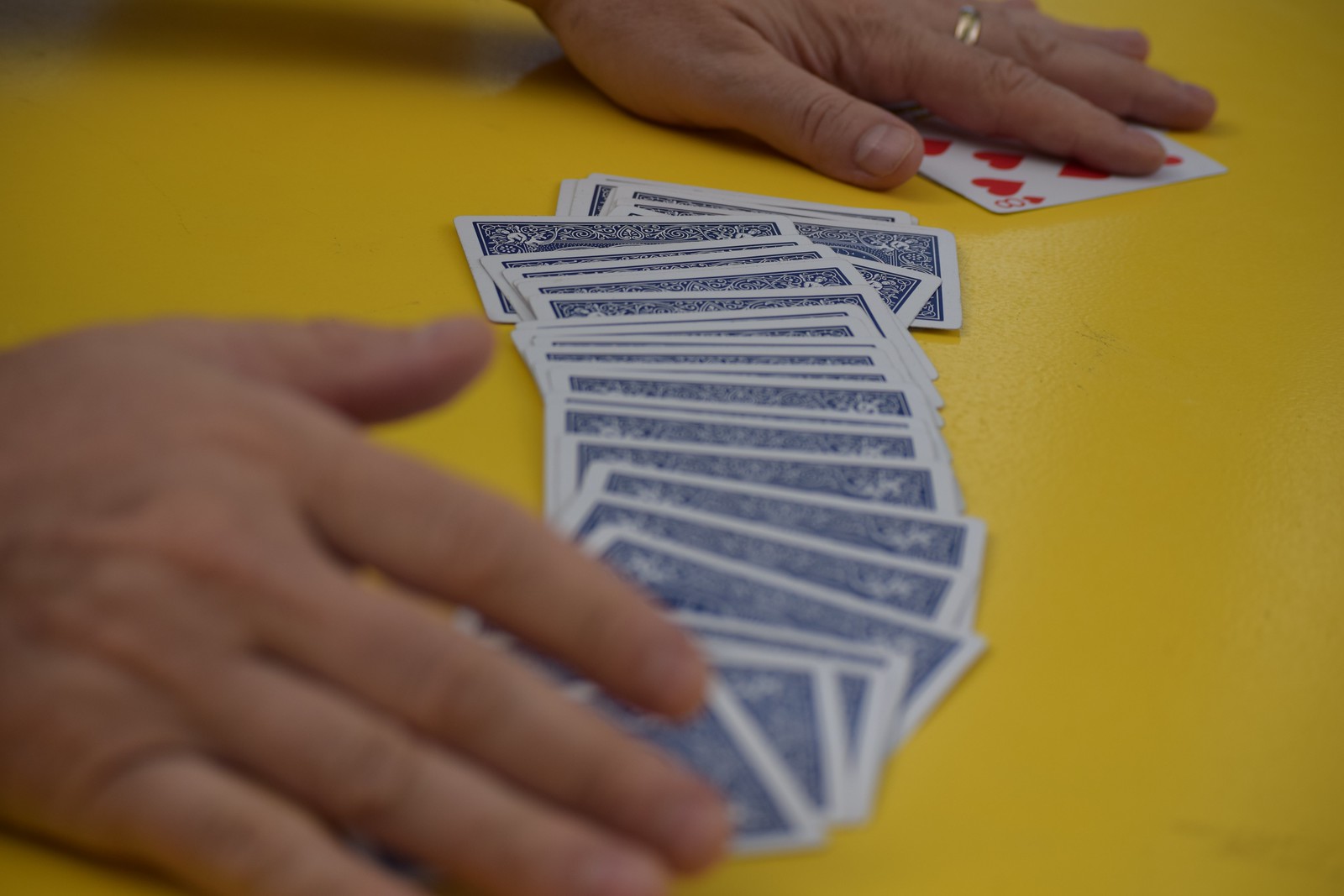This photograph captures a dramatic moment in a card game or a magic trick. A neatly spread deck of standard playing cards, facing down, occupies the center of the image. The cards showcase a classic navy blue paisley design with a thick white border. The scene is set against a vibrant yellow surface that contrasts strikingly with the dark colors of the cards.

Two hands, appearing to belong to a white person, dominate the composition. The left hand, adorned with a gold ring on the middle finger, hovers above the deck. Its index finger points directly across the middle of the eight of hearts, indicating a moment of action. This hand exhibits a slight blur, suggesting motion as if it's just finishing the elegant spread of the deck.

The right hand rests at the end of the spread, stabilizing the cards and framing the tableau. The precise arrangement of the cards and the careful placement of the hands imbue the image with a sense of skill and anticipation, capturing the viewer's interest and curiosity.